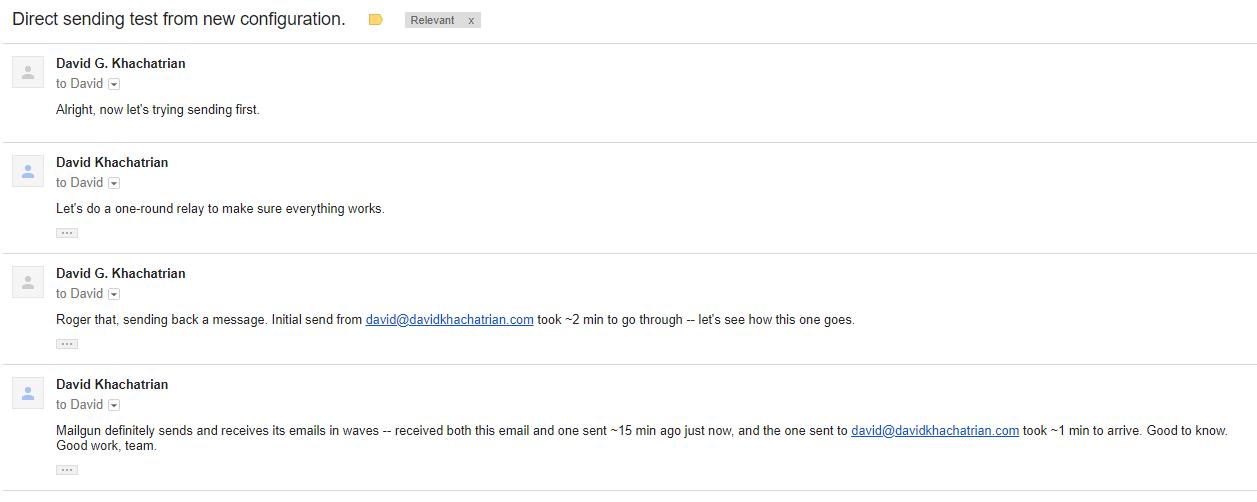This is a detailed screenshot from an unidentified web page showcasing a test of direct email sending from a new configuration. At the top, the title reads "Direct Sending Test from New Configuration" with a prominent yellow arrow pointing to the right. Below, there is a gray rectangle labeled "Relevant," with a small 'X' icon situated on the far right of this box.

The content features a series of email exchanges:

1. David G. Kachatrian to David: "Now let's try sending first."
2. David Kachatrian to David: "Let's do a one-round relay to make sure everything works."
3. David G. Kachatrian to David: "Roger that. Sending back a message."
4. Notes from David mention that the initial send from David@DavidKachatrian.com took around two minutes to go through. This message references the observation: "Mailgun definitely sends and receives its emails in waves. Received both this email and one sent 15 minutes ago just now," highlighting that the message took one minute to deliver.

The screenshot is described as being wider than it is tall and devoid of any photographic elements, people, or animals. The textual content is strictly related to the operational testing of email functionality, reflecting a technical behind-the-scenes dialogue among team members to ensure the smooth operation of their email system. The message concludes with an encouraging "Good work team."